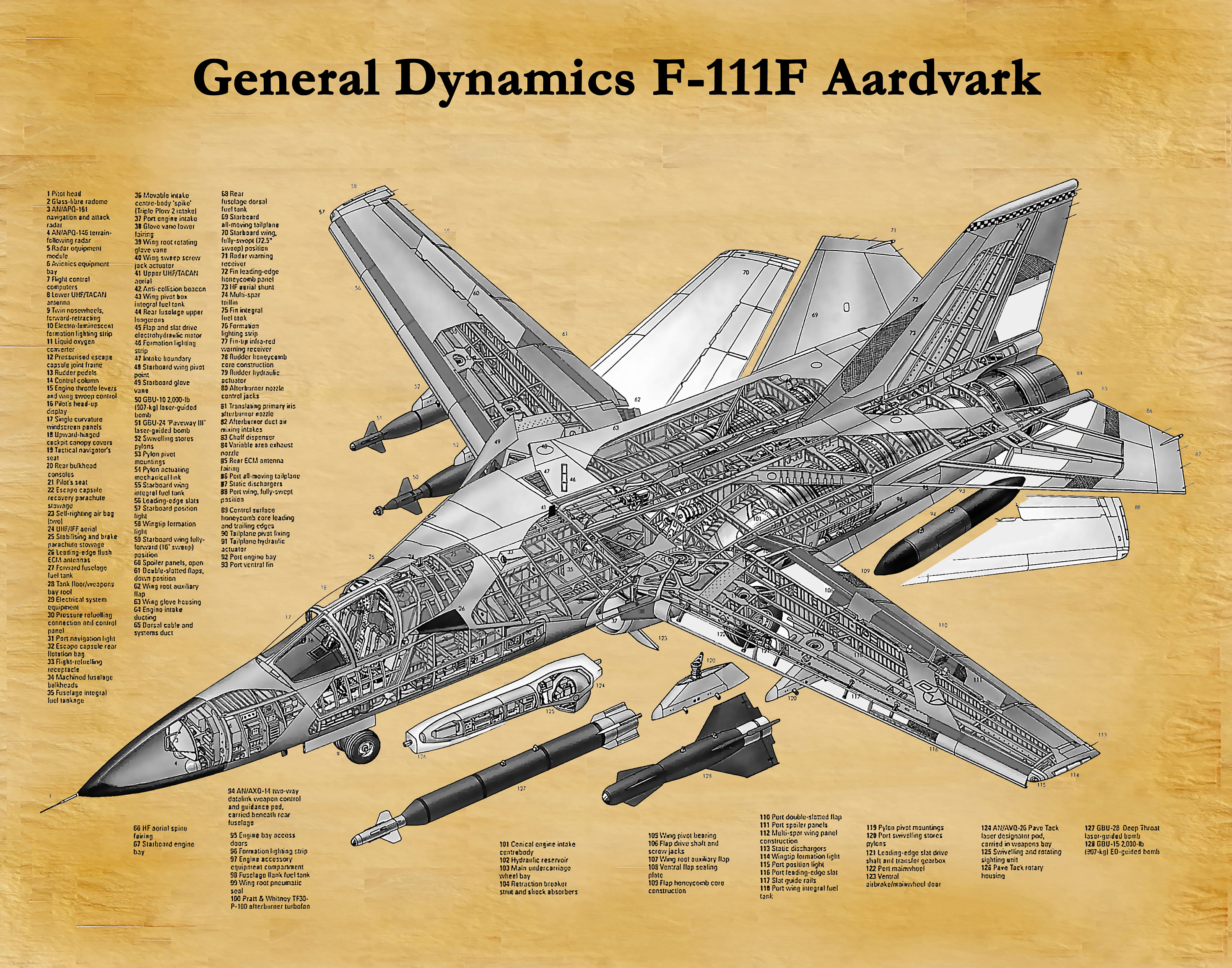This is a remarkably detailed poster of the General Dynamics F-111F Aardvark military aircraft. The top of the poster prominently features the plane's name in dark black letters, "General Dynamics F-111F Aardvark," set against a light golden-brown background that could be faux wood. Central to the poster is an intricate cutaway diagram of the F-111F, showcasing the plane's structural steel elements, including the wings and tail section. The illustration is meticulously annotated with over 120 numbered notations identifying each part of the aircraft, though the text is minuscule and challenging to read. Accompanying the plane are several missiles, indicating its role as a fighter plane. The diagram stretches across the poster with additional components illustrated towards the bottom and sides, reinforcing the comprehensive nature of this presentation, likely designed for detailed technical analysis in a meeting or a professional setting. The entire display, rendered in black, white, and shades of gray, highlights the complexity and sophistication of this military aircraft.